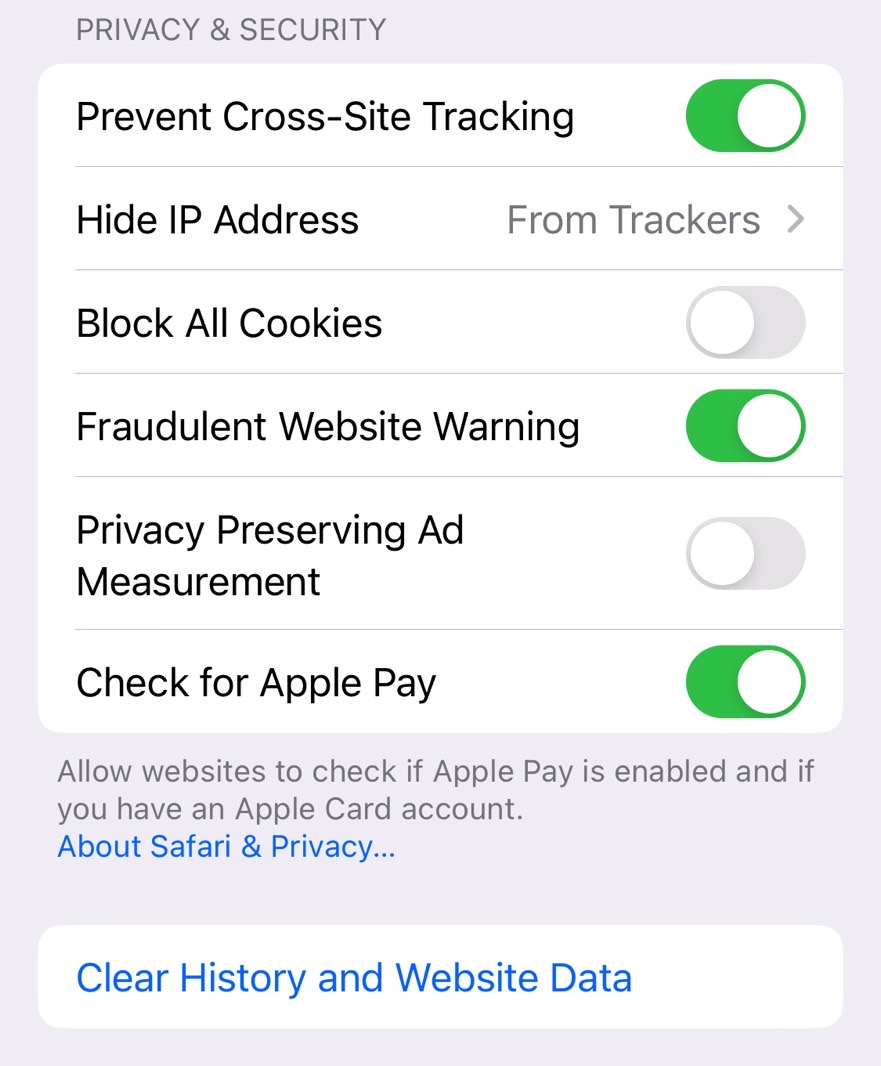This image shows the Privacy and Security settings screen for the Safari web browser. The settings displayed include:

1. **Prevent Cross-Site Tracking**: Enabled to stop information from being shared across different websites.
2. **Hide IP Address**: This option is not activated, though it suggests users might want to hide their IP address from trackers.
3. **Block All Cookies**: Disabled, enabling the use of most websites which require cookies for functionality.
4. **Fraudulent Website Warning**: Enabled, providing alerts for potentially dangerous sites.
5. **Privacy-Preserving Ad Measurement**: Disabled, meaning ads are not calibrated to preserve privacy in this user's configuration.
6. **Check for Apple Pay**: Enabled, allowing websites to verify if Apple Pay is available and if the user has an Apple Card account.

Additionally, there is an informational section titled "About Safari and Privacy," and a button at the bottom labeled "Clear History and Website Data," which allows users to erase their browsing history and data.